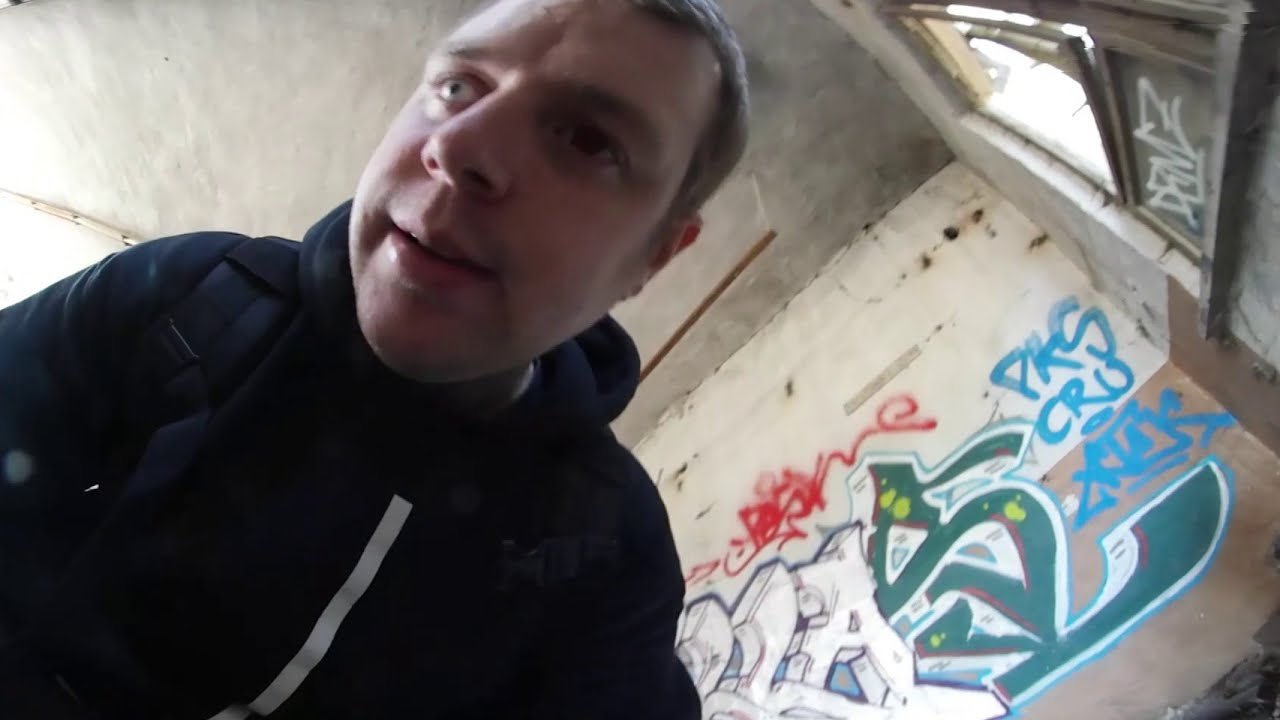The image portrays a young white male dressed in a dark hoodie with a distinctive white stripe running down the center, indicative of a zippered design. He has short hair, potentially brown or blonde, and appears to be capturing a photo of himself using a fisheye lens, giving the scene a distorted, angled perspective. His gaze is directed away from the camera, adding a natural, candid element to the shot. In the background, he stands inside what seems to be an abandoned, dilapidated building with a grungy aesthetic.

The building's interior features walls covered in a mix of white, tan, and concrete gray hues, heavily adorned with vibrant graffiti. Prominent among the colorful graffiti are large green, blue, and red letters, with a noticeable white lettering that resembles "LLA" to the right side. The graffiti includes varied imagery and symbols, with small yellow splotches accentuating the chaotic art. A window located in the top right of the image allows sunlight to stream into the room, contrasting with the dim, ambient light from the ceiling. The overall scene captures an urban, gritty atmosphere, with the young man leaning slightly to the right, his presence offset by the disarray of the graffiti-laden surroundings.